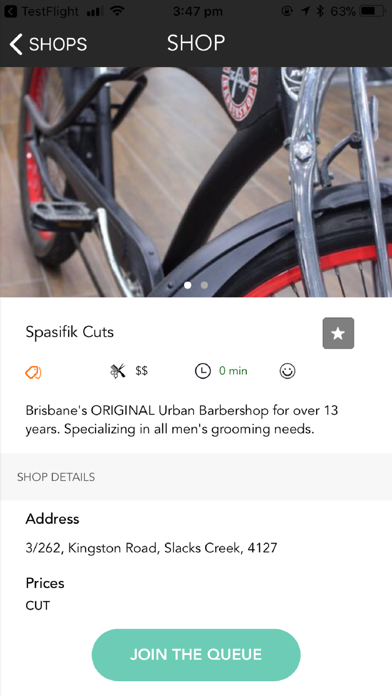**Caption:**

This screenshot showcases a mobile app interface, potentially related to cycling or a barber shop. The top overlay displays the device's status bar, including a Chrome app indicator, Test Flight label, signal strength, Wi-Fi status, time (3:47 PM), Bluetooth icon, and battery level (63%). Below the status bar, a navigation arrow beside the word "Shops" is visible, with "Shop" prominently displayed in the center.

A high-quality photo of a bicycle's frame dominates the screen. This close-up focuses on the bike's front forks, red rims, chain guard, pedals, and back tire, all set against an elegant dark brown hardwood floor. However, the top of the bike and the seat are not visible.

Beneath the image, the text "Specific Cuts" (stylized as "S-P-A-S-I-F-I-K Cuts") appears, suggesting a unique branding. Various icons accompany this text: a star, a price tag icon, scissors with a comb, and a smiley face, implying a service or rating system. The icons display two dollar signs and indicate a zero-minute duration.

Further description reads: "Brisbane's ORIGINAL urban barber shop for over 13 years specializing in all men's grooming needs." This captures the essence and legacy of the business. Additional details include the shop address: "3-262 Kingston Road, Slacks Creek, 4127." Below this, text for "Prices and Cuts" offers no additional information. At the very bottom is a prominent light green button labeled "Join the Queue," inviting users to get in line for services. 

This detailed caption encapsulates the visual and textual elements within the screenshot, highlighting both its apparent cycling theme and its unexpected barber shop context.